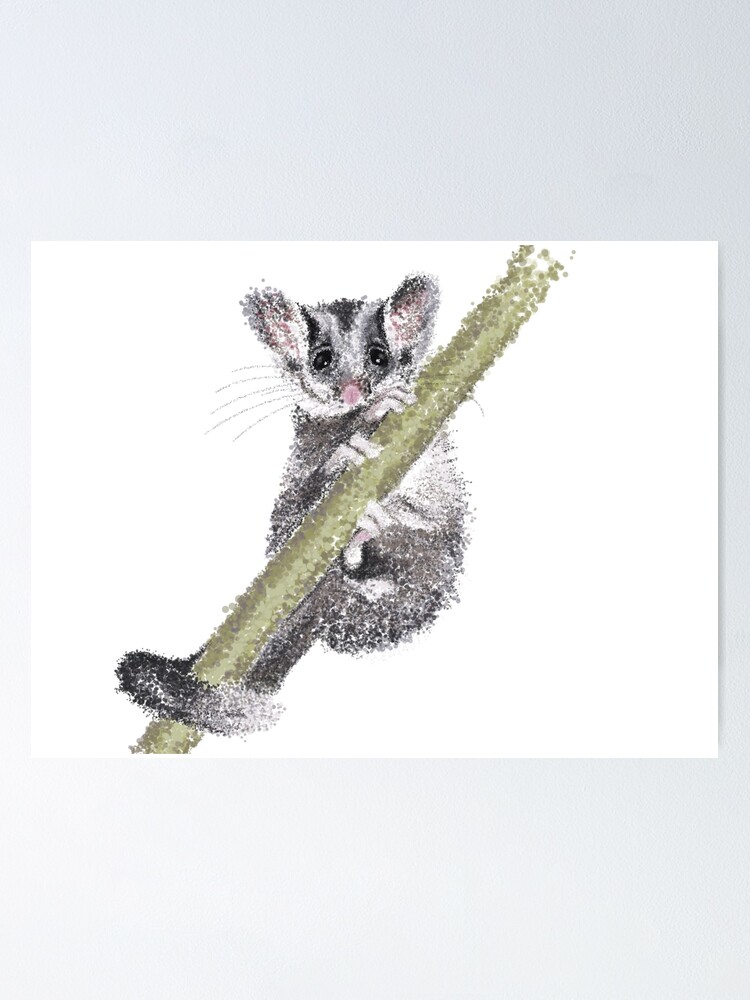The image is a detailed art print of a small, mouse-like creature that resembles a chinchilla or possibly a bush baby. The artwork is crafted using a stippling technique, involving thousands of tiny dots that give it a textured, splotchy appearance. The creature is clinging to a dusky green branch or blade of grass, with its long, fluffy tail wrapped around the branch for support. Set against a plain white or off-white background, the animal's features are distinctly gray, white, and flecked with bits of brown. It has two beady black eyes, a pink nose, and mini whiskers bristling from its face, with gray stripes spanning its forehead. The creature's ears and slight touches around its fingers show hints of pink. The animal appears to be peering directly at the viewer with a somewhat apprehensive expression, clutching the branch with claws and curled tail as though ready to react to its surroundings.